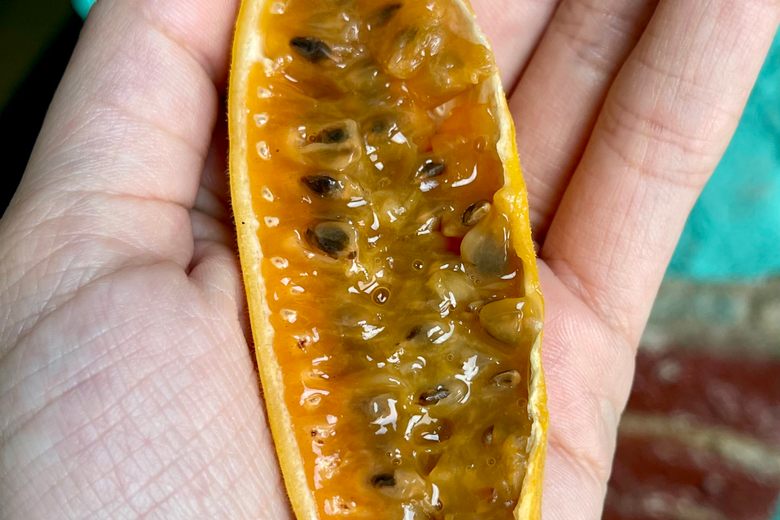In this detailed close-up photograph, a banana passion fruit is held in the open palm of a white man’s left hand. The image is remarkably clear, showcasing the intricate indentations of the skin on his hand. The fruit, with its shiny, orangish-yellow skin, has been sliced open to reveal a jelly-like center filled with dark brown to black seeds embedded in a gooey, brownish-orange gel. The background, blurred and composed of various shades of green, brown, blue, and gray, emphasizes the fruit and hand in the foreground, adding depth to the image. The oblong fruit has a rugged, bumpy texture on the rind, and the contrast between its vibrant exterior and the moist, slimy interior creates a visually appealing composition.